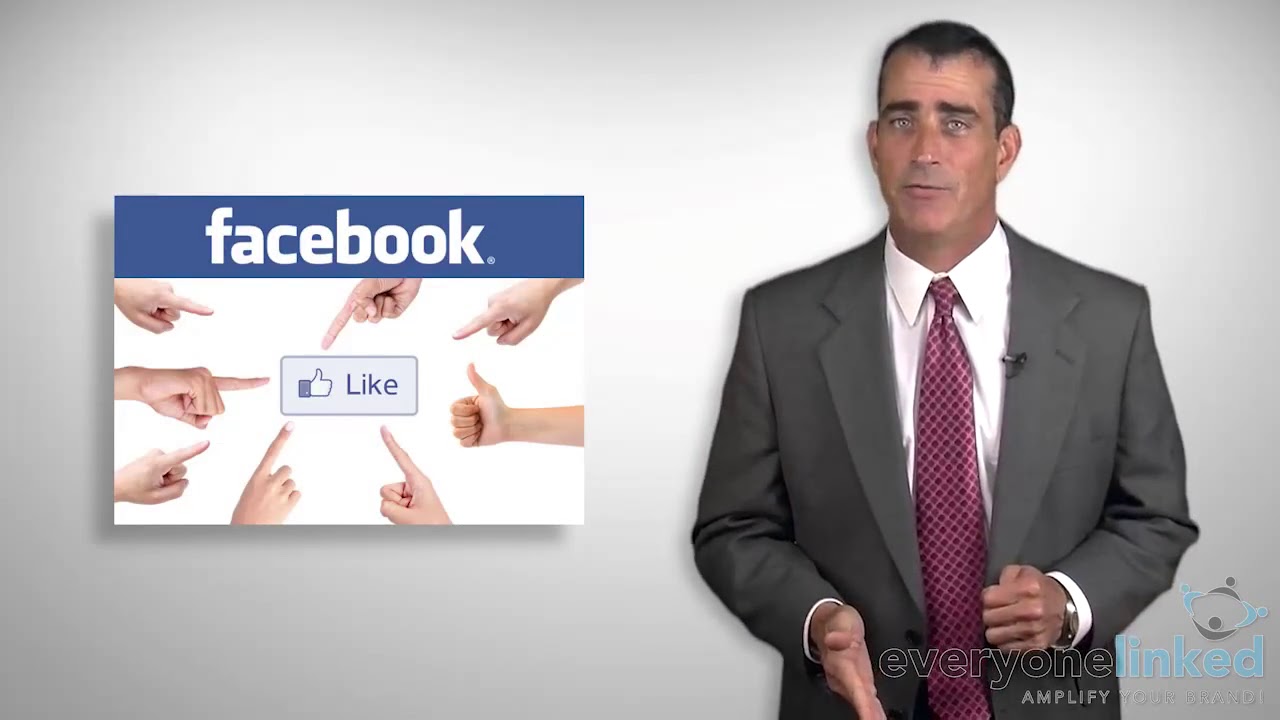The advertisement screenshot features a tan white man with dark hair, dressed in a dark gray business suit with a white or light pink dress shirt and a maroon tie adorned with a scale-like design. He is making a hand gesture, with his right hand clenched and extended forward, while his left hand, bearing a watch, is slightly open and facing forward. The man is looking directly at the screen. 

In the bottom right corner of the image, there is the phrase "everyone linked," with "everyone" in see-through text and "linked" in blue. Beneath this, the text "amplify your" is partially visible and appears semi-transparent.

To the left of the man, there is a square image resembling a poster with the word "Facebook" at the top in a blue banner. Surrounding this are numerous hands, some pointing fingers and others giving thumbs-up gestures towards a central "like" icon, representing the familiar Facebook "like" button.

Overall, the image appears to be promoting connectivity and engagement, possibly for a social media or professional networking service.